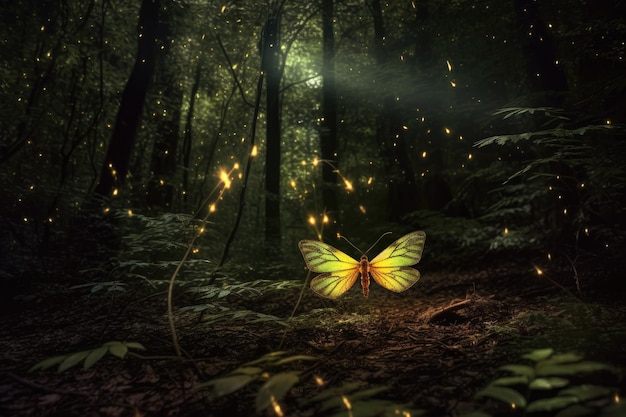This fantasy digital painting is set in a dark, densely wooded forest and captures a magical scene illuminated by a single break in the tree canopy at the top center. The faint light filters through the leaves, casting a gentle glow on the right-hand side of the image. Central to the illustration is a luminous butterfly, potentially self-illuminated or backlit, with a reddish-brown body and delicate, thin, outstretched antennas. The butterfly's wings transition from yellow near the body to a radiant neon green at the tips, giving it an ethereal quality as it flutters above a small forest clearing. Surrounding the butterfly are numerous fireflies, some leaving light trails, adding to the enchanting atmosphere. The forest floor below is brown and scattered with leaves, while the background is filled with indistinct but rich forestry, showcasing the vibrant, green foliage and the intricate details of the trees and bushes. The painting is devoid of any human presence, buildings, or mechanical objects, emphasizing its pure, natural beauty.